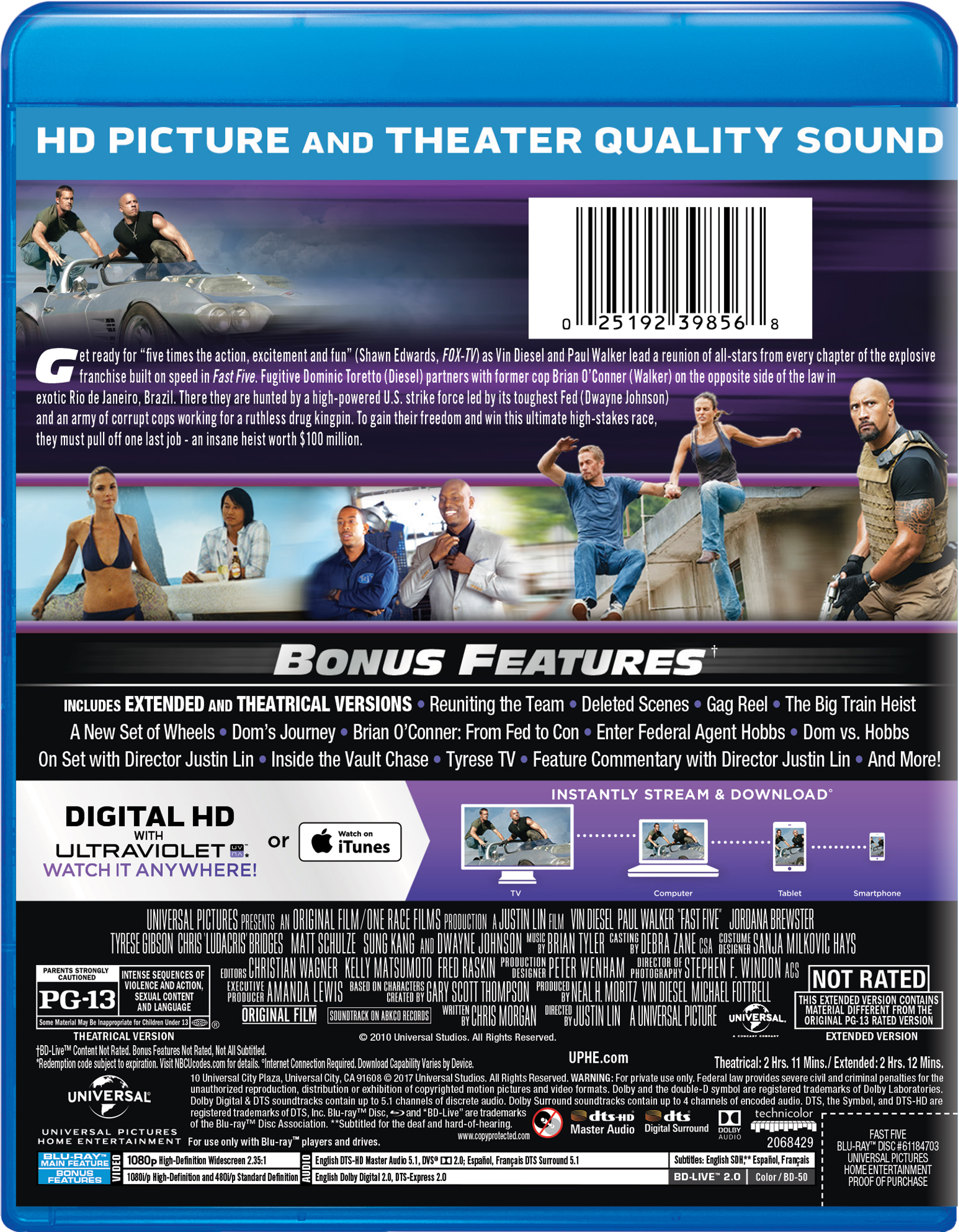This is the back of a blue DVD case with a multi-colored wrapper featuring shades of blue, purple, black, dark gray, and white. At the top, in bold white capital letters, it announces "HD PICTURE AND THEATER QUALITY SOUND". Below this, there's an image of two men in dark t-shirts inside a fast-moving silver car, appearing ready to leap out, likely from the "Fast and Furious" series. 

Next to the image is a synopsis that reads: "Get ready for five times the action and excitement as Vin Diesel and Paul Walker lead an all-star reunion in the explosive franchise built on speed. In 'Fast Five', fugitives Dominic Toretto (Vin Diesel) and Brian O'Conner (Paul Walker)..." The complete text is hard to decipher due to its small size.

Additionally, there is a barcode on the right. Underneath the synopsis, a strip displays scenes from the movie, followed by a bold "BONUS FEATURES" section listing special content. Below this, a white and purple strip highlights "DIGITAL HD WITH ULTRAVIOLET - WATCH IT ANYWHERE," promoting the digital viewing options.

Along the bottom edge, you'll find the movie’s rating, PG-13, and an array of technical and legal information, including production credits, audio and visual specifics, DVD format details, and FBI warnings. This extensive text and imagery layout, despite lacking a clear title for the movie, thoroughly conveys its high-action, star-studded nature, typical of the "Fast and Furious" series.